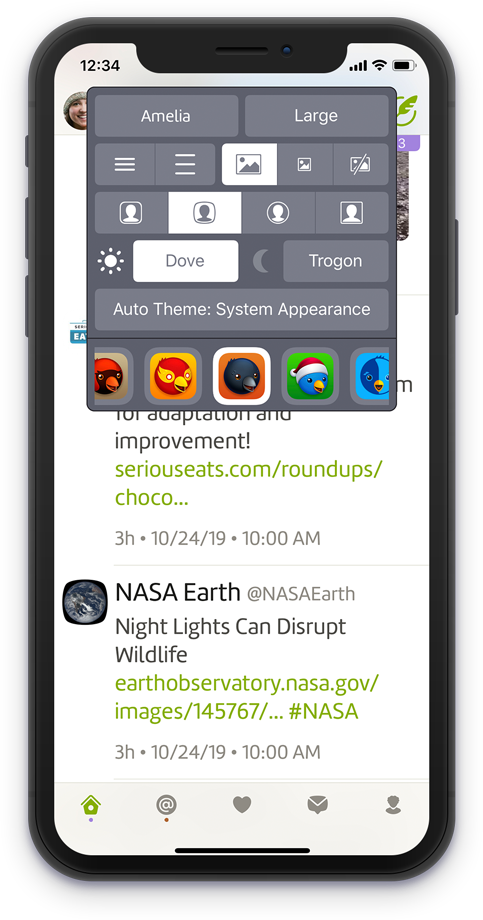This screenshot captured from a cell phone displays several interface elements and notifications. The time shown is 12:34, although it's not specified whether this is AM or PM. The phone's battery is nearly fully charged, and icons indicate both Wi-Fi and cellular signals are active.

At the top of the screen, two gray buttons are labeled "Amelia" and "Large." Below these, two buttons feature three lines each, one set is close together, and the other set is further apart. The interface also includes three boxes; the first contains a highlighted picture, the second has a smaller picture, and the third is empty and not highlighted.

Further down, there are icons representing different profile sizes: a small profile picture, a larger highlighted profile picture, a profile with a circle around it, and a profile with a square, which is not highlighted. Below these, a sun icon labeled "Dove" is highlighted, while a moon icon and the word "Trogon" are not highlighted.

The interface displays a section titled "Auto Theme: System Appearance." Beneath this section, there are images of birds resembling cardinals and penguins, some adorned with Santa Claus hats. 

Following this, a text section reads: "For adaptation and improvement. Seriousseats.com/roundup/chocolate..." This is timestamped "three hours ago, 10/24/19 at 10 a.m." 

Lastly, a picture of planet Earth is accompanied by the text: "NASA Earth @NASA Earth. Night lights can disrupt wildlife. Earthobservatory.nasa.gov/images."

This detailed summary highlights various interface elements and information presented on the phone screen.